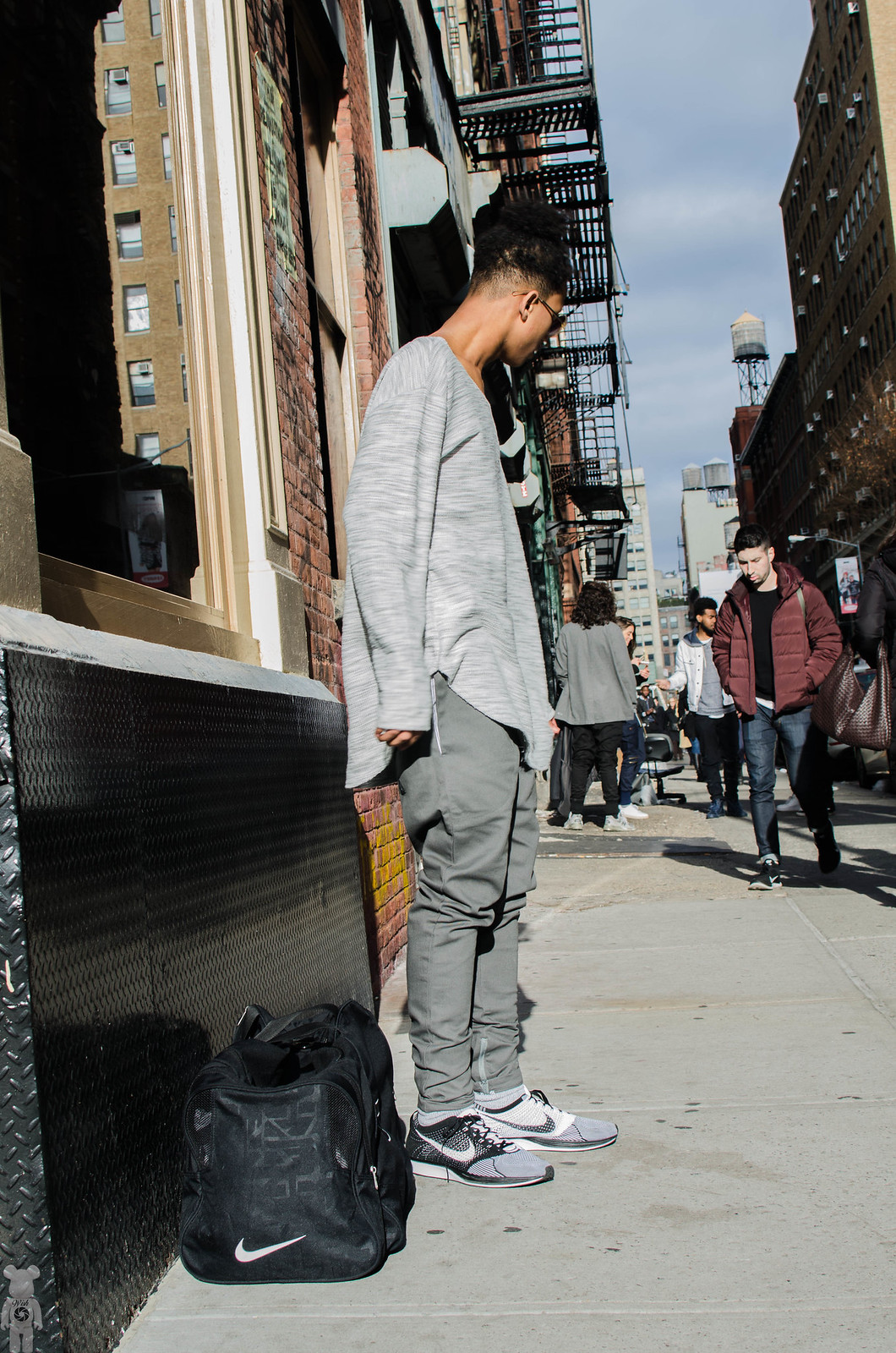The photograph captures a man with dark black hair and caramel-colored skin, standing on a sidewalk next to a building with reflective windows behind him. He is wearing a loose, long-sleeve t-shirt and dark gray or light gray trousers, paired with gray sneakers that feature black accents and the iconic Nike Swoosh logo. The man is also carrying a black Nike sports duffel bag, identifiable by the white Swoosh logo at the bottom. He has glasses on and is looking down at the sidewalk. Beside him, to his left, is a black backpack with another white Nike tick. 

In the background, various elements of an urban setting are visible, including fire escapes, tall buildings with water towers, and people walking along the gray sidewalk. Notably, a white man in a maroon puffy jacket and dark blue jeans is seen walking on the right side of the image. Additional figures, including some women and other men, can be observed further down the sidewalk. The image highlights a bustling city atmosphere with a mix of personal styles and movement.